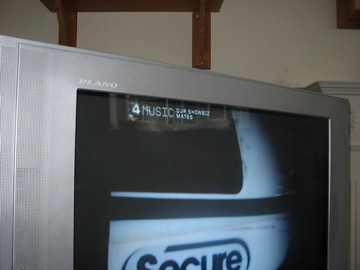The image is a close-up photograph of an old-style, dull, silver-bordered CRT TV screen in a room with white walls. The TV display shows a partial graphic in black and white, which reads "secure," though the full word isn't visible as the screen image is cropped. At the top left corner of the screen, the text "4 Music" is displayed. The wide gray border of the television has the word "Plano" inscribed in white letters. The television appears to be reflecting the front of a house or possibly a vehicle's side. Surrounding the TV, there's a wooden shelf attached to the white wall with visible supporting struts below it. The photograph captures only the top two-thirds of the TV, leaving the bottom part out of the frame. The layout suggests a room with a white balustrade visible to the right.